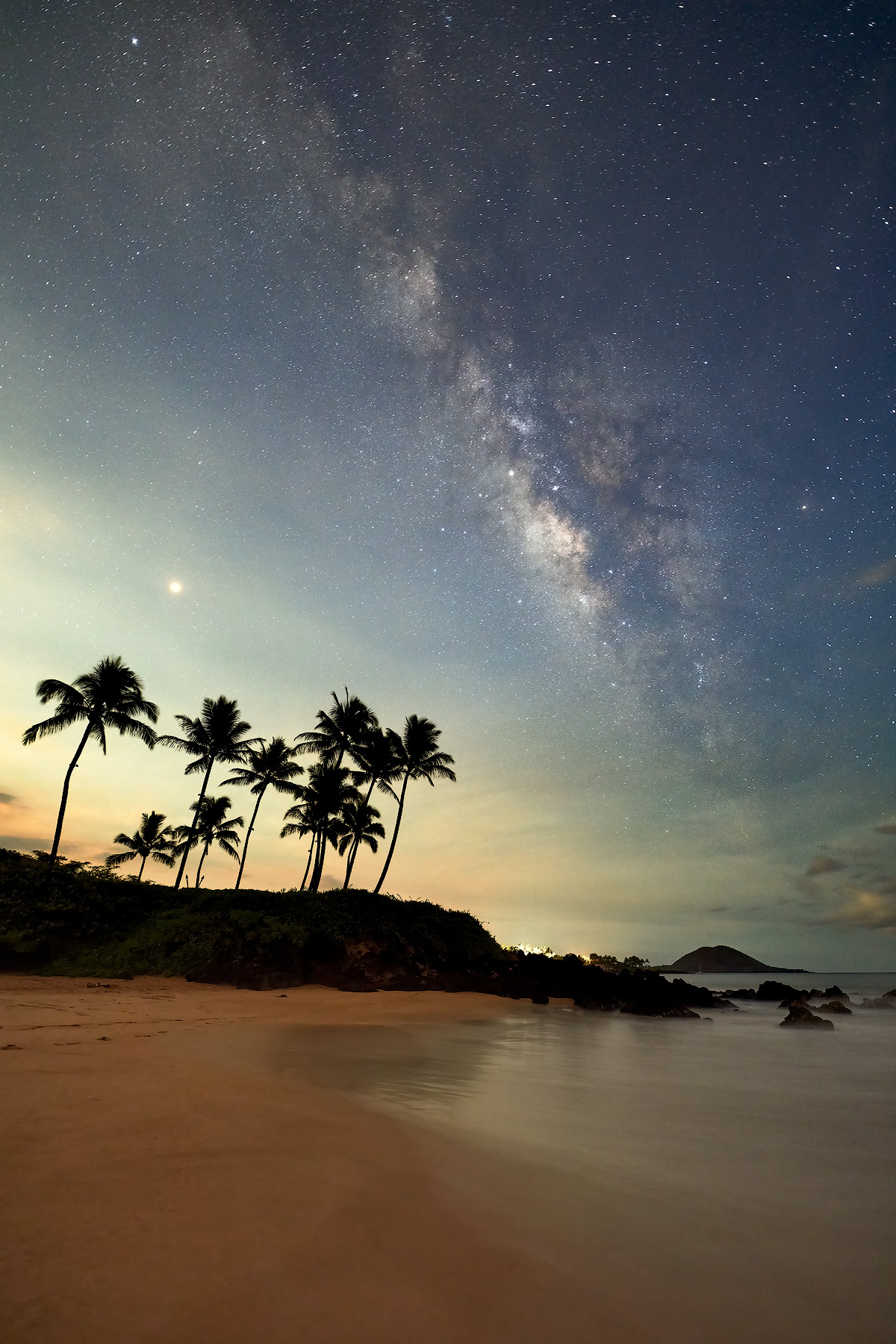This captivating photograph depicts a serene twilight scene on a tropical beach coastline. The composition is richly colored, with a tranquil ocean meeting deep reddish-brown sand. The water is calm, giving a sense of peaceful isolation. To the left, you can see a cluster of tall palm trees standing on a gently sloping hillside, their leaves appearing almost black against the backdrop of the setting sun. The sky is a mesmerizing blend of vivid hues, transitioning from a bright dark blue on the right to a softer baby blue on the left where the sun is setting.

Above, the night sky is illuminated by a spectacular display of stars, with the Milky Way visibly stretching from the middle right to the upper left. Gaseous clouds of stars add to the celestial spectacle, making the sky appear almost otherworldly. A distant outcropping or island can be seen far off in the horizon, adding to the depth of the landscape. This breathtaking scene captures the essence of a tropical paradise as day transitions into night, leaving the viewer longing to visit this stunning and tranquil place.